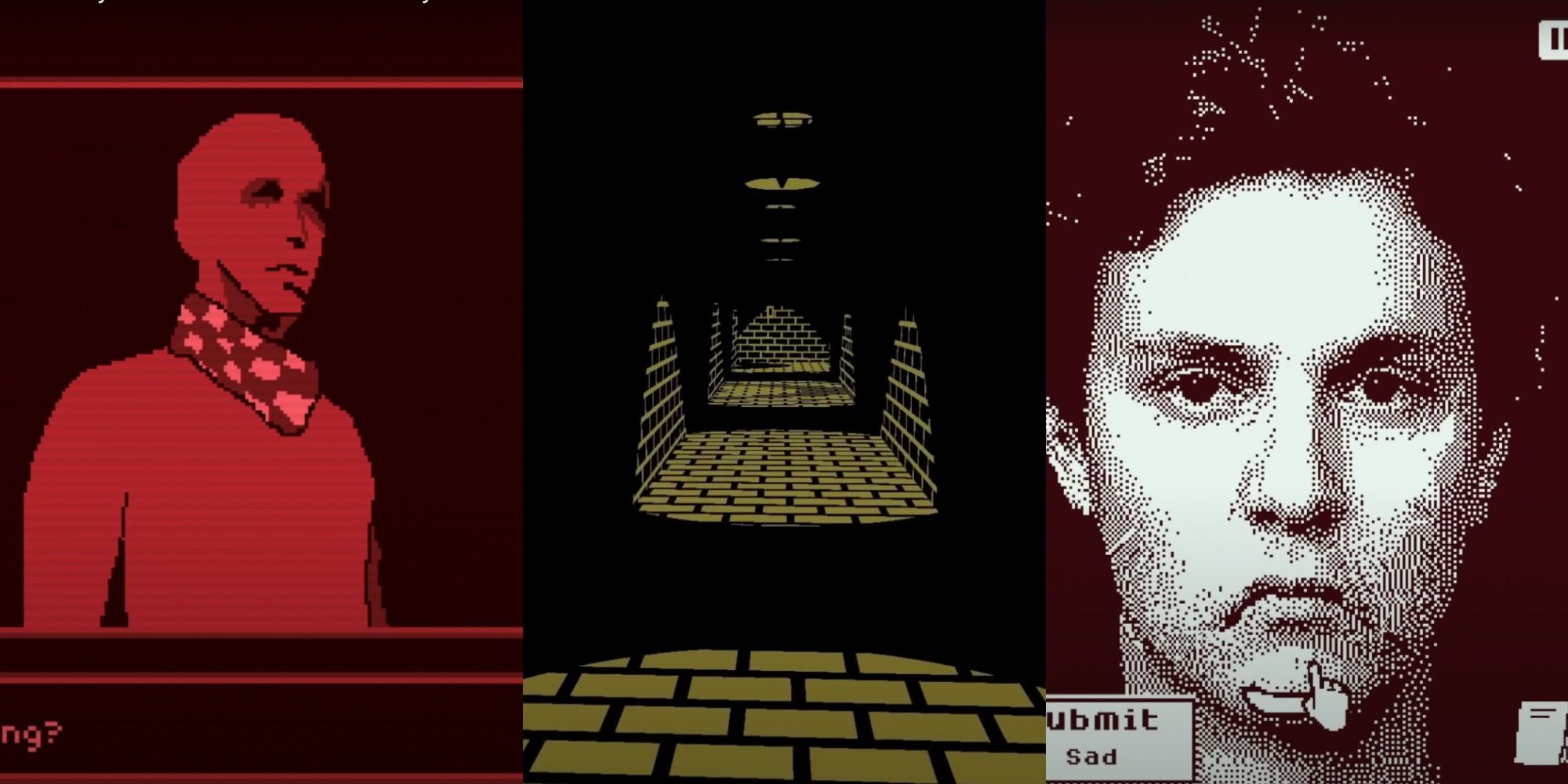The image is a triptych comprising three distinct panels, each with a unique, pixelated graphic reminiscent of old video games:

On the left, there is a red human figure set against a maroon background with red lines. This character, who appears to be bald, is adorned with a red and pink checkerboard scarf and positioned to look towards the right. The bottom of this panel features the cutoff text "NGP".

In the center panel, the scene resembles a classic video game like Wolfenstein, depicting a dark tunnel with green bricks and black mortar extending into the distance. The setting is stark, with a black background emphasizing the tunnel's depth.

The rightmost panel features a highly pixelated, black and white image of a man's face. The man has a frown and looks straight ahead. A mouse pointer icon is directed at his chin. There is text reading "UBMIT SAD", seemingly cut off, possibly suggesting the word "submit." The image retains a graphical, textured quality, dominated by black, white, and hints of maroon.

Overall, the composite image evokes a strong sense of early video game aesthetics through its pixelated designs and simplified color palette.